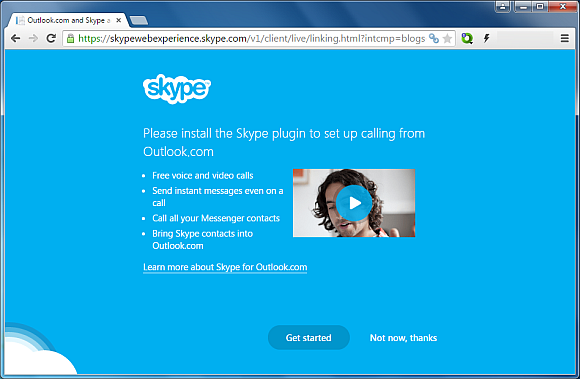The image is a computer screenshot of a Skype page with a blue background. In the top left corner, the browser tab is visible, directly below which is the HTTPS web address of the page. Beneath the web address, there is a Skype logo with the word "Skype" in blue letters outlined in white. 

The main prompt on the page reads, "Please install the Skype plugin to set up calling from outlook.com." Below this prompt, there are four bullet points in white text, listing the features of the Skype plugin:
- Free voice and video calls
- Send instant messages even during a call
- Call your messenger contacts
- Bring Skype contacts into Outlook

To the right of the bullet points, there is an embedded video preview with a play button, featuring an image of a man with long brown hair. Below the bullet points and the video preview, there's additional text that reads, "Learn more about Skype for outlook.com."

At the bottom of the section, there are two buttons: a blue, pill-shaped button that says "Get Started" and a grey button that says "Not now, thanks." In the bottom left corner of the screenshot, there's a small partial white cloud.